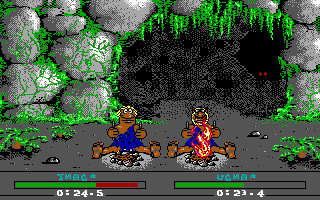The image is a screen capture from a retro-styled video game with graphics resembling the 8-bit or 16-bit era, possibly from the SNES era. It depicts two cavemen named Thag and Uka, identifiable through their health bars at the bottom of the screen, one of which shows their health partially depleted with a mix of green and red in the bar, and specific time indicators beside them. The scene shows the cavemen wearing blue, spotted outfits, sitting with their legs stretched out in front of them, each holding utensils and facing a campfire situated between their legs. One fire is extinguished while the other burns brightly. They sit outside a large stone cave with spooky red eyes peering from a dark crevice in the background. There are green plants, including moss and possibly small palm trees, growing around the rocks and on either side of the scene, adding to the prehistoric ambiance.